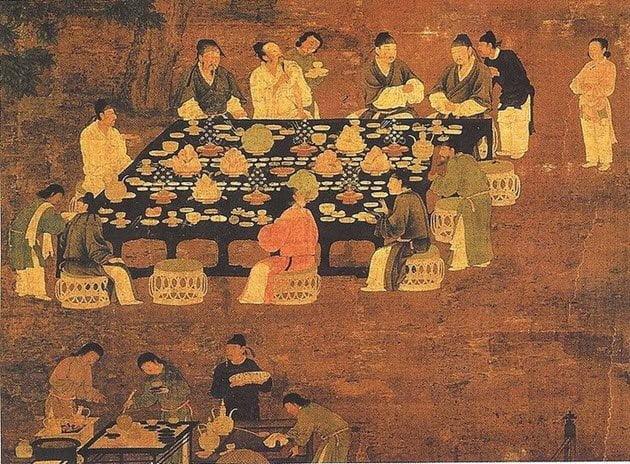The artwork portrays an ancient Asian dinner scene, richly detailed and predominantly rendered in brown hues. At the heart of the square canvas is a large black table, laden with a variety of plates and trays of food. Surrounding the table are approximately 15 individuals, men and women alike, dressed in robe-like gowns of varied colors—some white, black, and brown, with one notably in orange or red. These figures are seated on wicker baskets with tan or green cushions, adding texture to the scene. Some of the individuals are seated, while others are standing, including a woman in the upper right corner who stands apart with her arms folded. In the foreground, people can be seen engaging in cooking activities with various instruments. The background of the image is characterized by earthy tones of brown, with a touch of green from tree branches in the upper left corner, evoking a rustic outdoor setting with dirt, ground, or rocks. The overall composition, potentially executed in watercolor or oil-based paint, captures the essence of communal dining in an ancient Asian milieu.